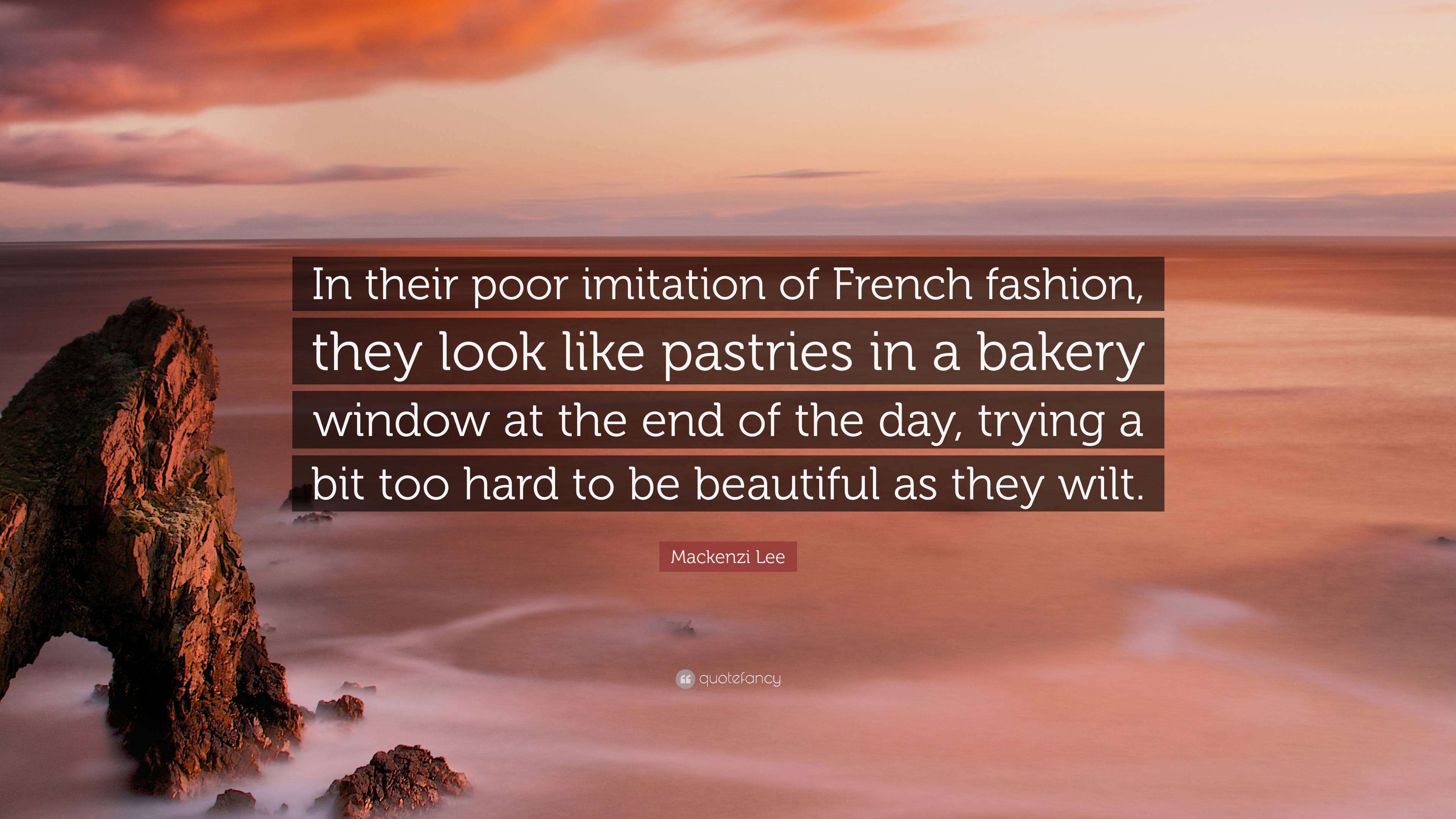The poster features a striking landscape that closely resembles an otherworldly terrain, reminiscent of a Martian landscape with its prominent reddish hue. Dominating the scene is a large, dramatic geological formation—a massive rock with a hollowed-out bottom—set against a backdrop where even the sky is a vibrant red. Intriguingly, the sky blends into a purple horizon, accentuated by a single red cloud that brightens towards the right side.

In the center of the image, a series of black and red bars with orange designs create a semi-transparent overlay that does not completely obscure the view of the stunning vista. Thin, dark lines are interspersed among these bars and carry a quote in white text: "In their poor imitation of French fashion, they look like pastries in a bakery window at the end of the day, trying a bit too hard to be beautiful as they wilt." Attributed to Mackenzie Lee, the quote adds a whimsical yet poignant reflective touch to the visual spectacle.

Additional elements include a grey circle with indistinguishable white symbols inside it, positioned near another text overlay to the right that simply reads "Fancy." The poster masterfully blends geological majesty with introspective commentary, creating an inspirational piece that evokes both wonder and contemplation.